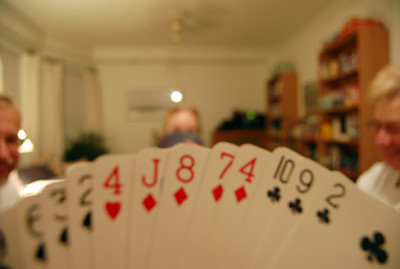In the foreground of the image, a hand of playing cards is splayed out, obscuring parts of the view but showing several cards: the six, three, and two of spades; the four of hearts; the jack, eight, seven, and four of diamonds; and the ten, nine, and two of clubs. The background of the photo is blurred, revealing a room with slightly ivory-hued white walls and ceiling. On the left side, curtains hang down, adding a touch of elegance. To the right, two bookcases brimming with books suggest a well-read household. Behind the cards, two men can be seen on either side of the cardholder. The man on the right sports a blondish hue of hair, glasses, and a mustache. The man on the left has darker hair and also appears to have a mustache. Directly opposite the cardholder, another individual is partially visible, but their features are obscured by the raised cards, making it unclear if they are male or female.